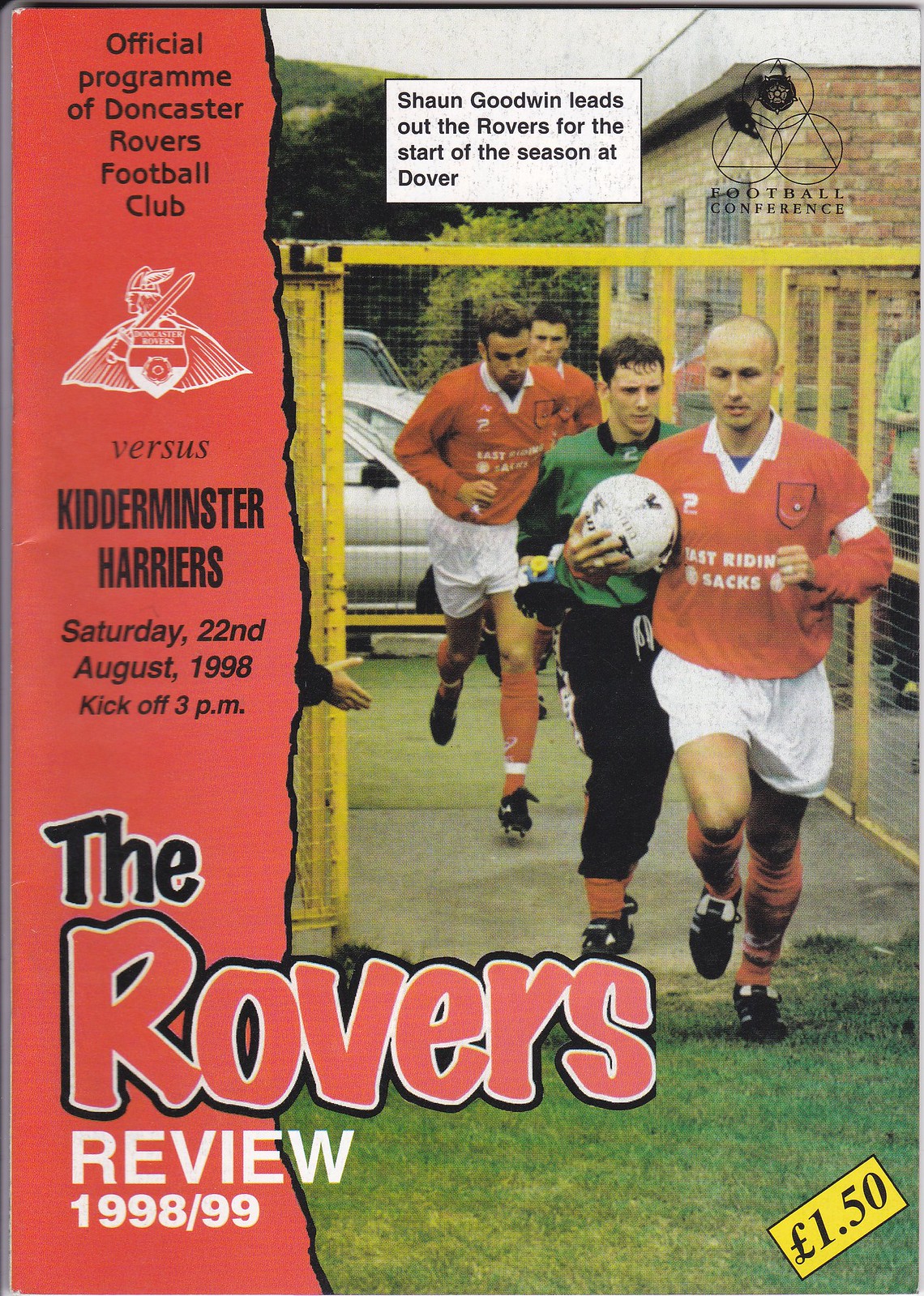The image is a game day program cover for the Doncaster Rovers Football Club. Dominating the left side, a red vertical bar with a torn right edge features most of the text. At the top, it reads "Official Program of Doncaster Rovers Football Club," accompanied by an emblem depicting a Viking with wings, sword, and shield. Below, in black text, it states "Versus Kidderminster Harriers, Saturday, 22nd August 1998, kickoff, 3 p.m." The title "The Rovers Review 1998-99" is prominently displayed in large white and red text at the bottom left. On the right side, an action photo captures the Rovers' players—three in red jerseys and the goalie in a green jersey—running onto a grassy field. Above the photo, a caption reads, "Sean Goodwin leads out the Rovers for the start of the season at Dover." A small yellow badge at the bottom right indicates the price, marked as £1.50.